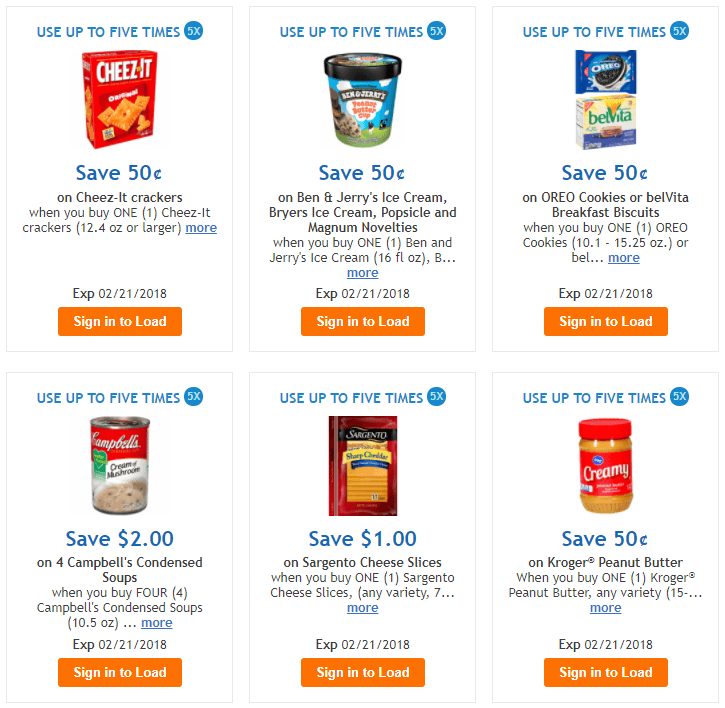This is a detailed screenshot from a coupon app or website, presented on a white background and organized into two rows of three vertical rectangles. Each rectangle contains a specific coupon offer.

In the first rectangle of the top row, there is a voucher for Cheez-It crackers. A prominent red box displays an image of a box of Cheez-Its in the center. Above the image, the text indicates that this coupon can be used up to five times. The coupon offers a savings of 50 cents when you purchase one box of Cheez-It crackers. Located below this information is the expiry date of February 21, 2018, along with an orange rectangular "Sign In" button. Clicking this button will load the coupon, prompting you to sign in to the app or website.

The second rectangle features a coupon for Ben & Jerry’s ice cream, also offering a savings of 50 cents and usable up to five times. 

The third rectangle of the first row offers a similar deal: 50 cents off when purchasing Oreo cookies or Belvita biscuits, with the same usage limit of five times.

All coupons in the first row share the same expiry date and include the orange "Sign In" button to load the coupon.

In the bottom row, the first rectangle contains a coupon to save $2 on four Campbell’s condensed soups.

The second rectangle offers a $1 savings on Sargento cheese slices.

The final rectangle provides a 50-cent savings on Krager peanut butter.

Each coupon in the bottom row also features the same "Sign In" button to load the coupon into your account.